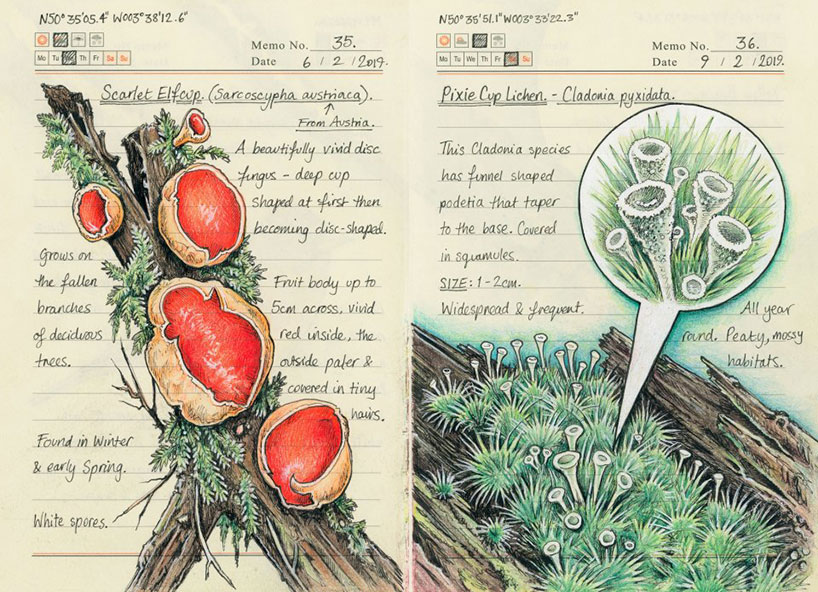The image depicts two pages from a nature notebook, each featuring detailed illustrations and descriptions of different plant species. On the left page, there's a detailed drawing titled "Scarlet Elf Cup" (with its scientific name included) showcasing a broken branch with vivid, deep red cup-shaped fungi growing on it, surrounded by paler, hairy exteriors. The descriptive text on this page notes that this disc fungus, which evolves from cup-shaped to disc-shaped, appears in winter and early spring and grows on fallen branches of deciduous trees. It distinctly mentions the fungal fruit body's size, which can reach up to five centimeters across, and highlights the presence of white spores.

On the right page, the notebook presents a labeled illustration of "Pixie Cup Lichen" (also with its scientific name), which features feathery green growths emerging from wood. These are described as funnel-shaped podetia covered in tiny leaf-like structures called squamules, with sizes ranging from one to two centimeters. The text notes that this Cladonia species is widespread, frequent, and thrives year-round in peaty, mossy habitats. Additionally, there's an inset magnified image focusing on the tubular growths for better detail.

Each page's information is meticulously handwritten on lined paper, providing an informative and visually appealing presentation of these fascinating natural specimens. The notebook also includes various memo numbers and dates related to the observations, namely June 2, 2019, and September 2, 2019, corresponding to the Scarlet Elf Cup and Pixie Cup Lichen, respectively.